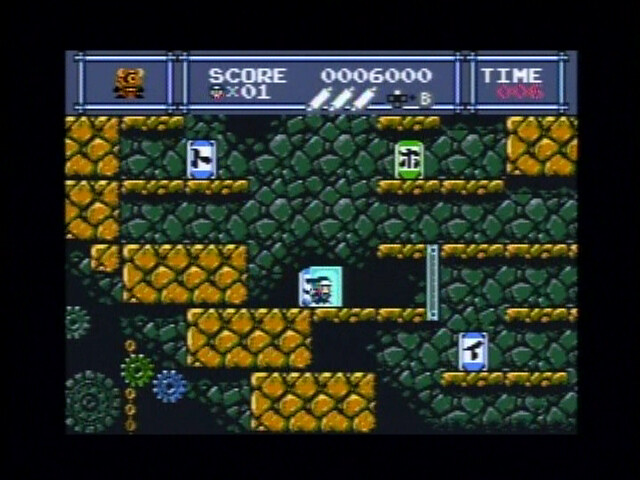The image displays a video game screen with a distinct artistic design. The background predominantly features a combination of green and yellow bricks arranged in multiple levels. The bricks are irregular in shape, resembling natural stonework rather than typical rectangular bricks. The scene unfolds across at least five levels stacked vertically from the bottom of the image.

Notably, the yellow brick surfaces are adorned with various playing card-like elements in shades of blue, green, black, and white. Some cards bear characters in an unfamiliar language, while one card appears to depict a multicolored face pattern of white and blue. The top of the screen features a blue border that contains detailed player information, providing functional context within the game.

This entire in-game scene is encased within a black border, framing the visual display neatly. The overall aesthetic suggests a thoughtful blend of traditional and imaginative design elements, contributing to an immersive gaming experience.